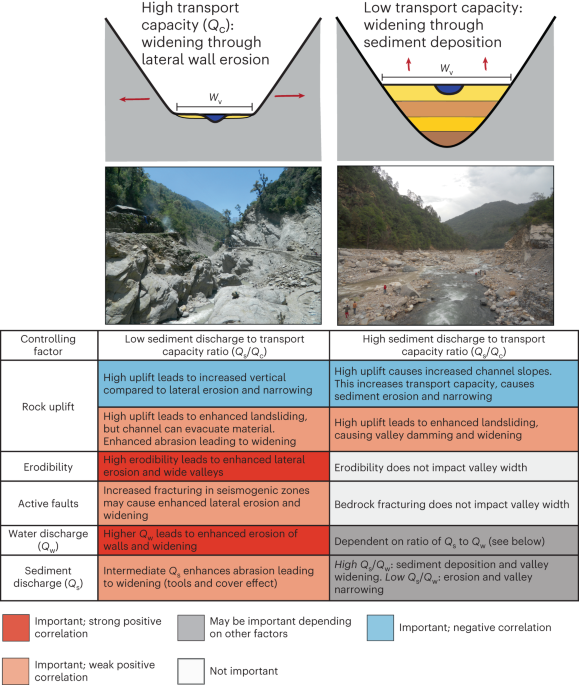This image, likely from a scientific presentation or book on sediment transportation, features a detailed comparison of high and low sediment transport capacities and their effects on landscape morphology. 

At the top, black font labels the contrasting processes: "High Transport Capacity, Widening Through Lateral Wall Erosion" on the left, and "Low Transport Capacity, Widening Through Sediment Deposition" on the right, with diagrams illustrating each scenario. The left diagram shows a valley with lateral wall erosion in a rocky riverbed, flanked by trees and hills, while the right diagram depicts a similar landscape with a river, highlighting sediment deposition.

Below these diagrams, a comprehensive table takes up the bottom section. The table is six rows by three columns, categorizing critical factors influencing sediment transport: "Controlling Factor," "Low Sediment Discharge to Transport Capacity Ratio," and "High Sediment Discharge to Transport Capacity Ratio." The rows are labeled with key controlling factors: "Rock Uplift," "Erodibility," "Active Faults," "Water Discharge," and "Sediment Discharge." Each cell within the table contains specific data, with color-coding indicating the significance of correlations — red for strong positive correlation, blue for important negative correlation, gray for potentially important factors, light red for weak positive correlation, and white for non-important factors. This detailed caption showcases not only the visual but also the analytical aspects of sediment transport phenomena.